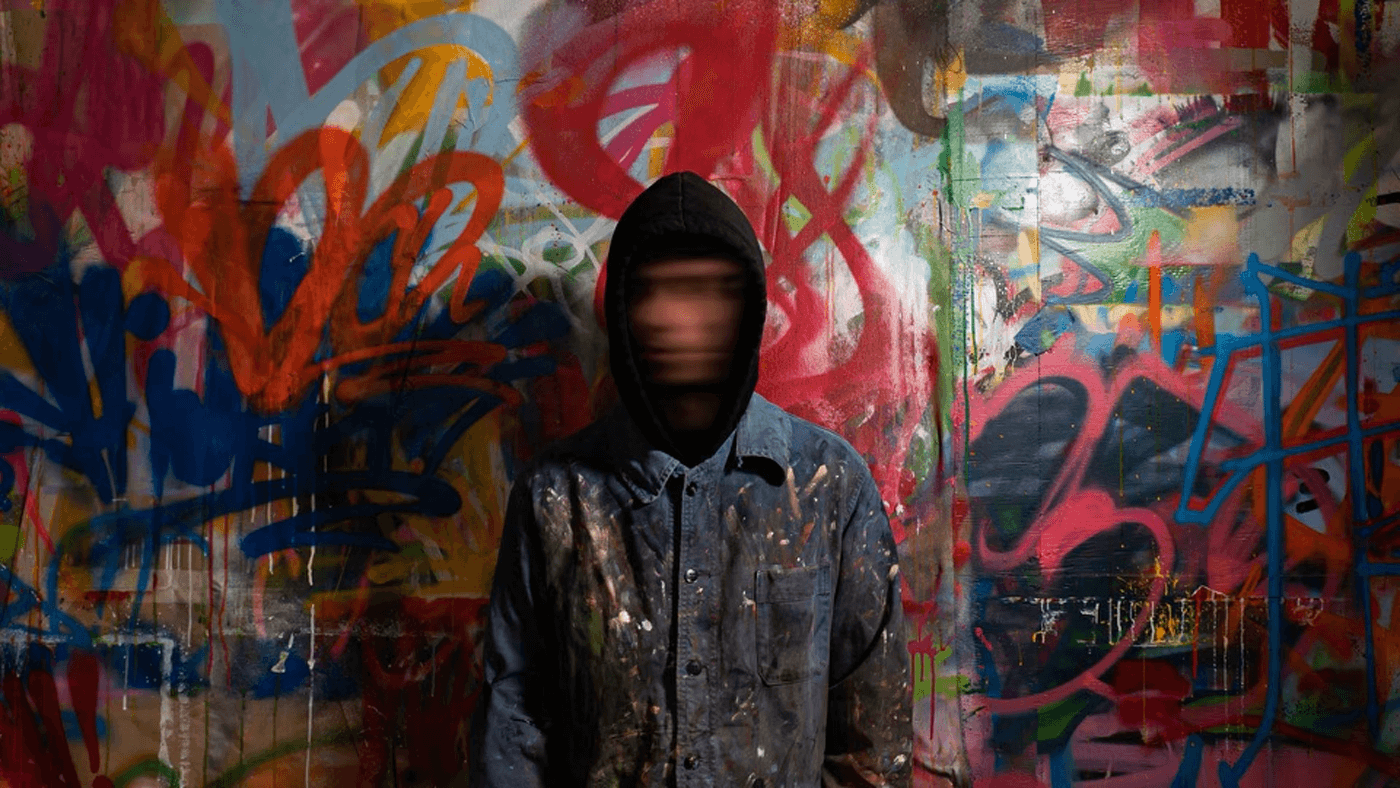The image depicts a horizontally aligned rectangular photo featuring a man standing against a vibrant graffiti wall. The background is a kaleidoscope of swirling colors, including shades of red, blue, pink, white, gray, black, green, and magenta. The graffiti consists of abstract shapes, swirls, and random patterns with no discernible figures, giving an impression of layers upon layers of paint. A faint number five is noticeable among the chaotic artistry.

In the center of the picture stands a man, partially obscuring the graffiti. He is dressed in a black hoodie under a blue denim jacket that is heavily splattered with various colors of paint, suggesting he might be a painter immersed in his work. His face is blurred, likely from motion, creating an effect that conceals his identity and adds a dynamic element to the image. The intricate mix of colors in the graffiti and the paint on his jacket blend harmoniously, reinforcing the urban and artistic theme of the photo.